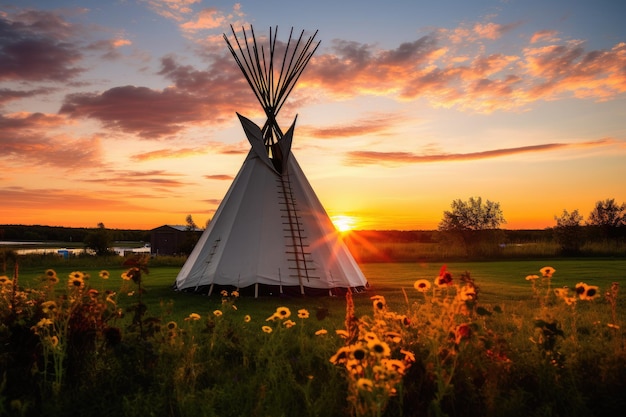The image showcases a modern, stylized teepee set in the midst of a lush, expansive grassy field at sunset. Dominating the foreground is a vibrant expanse of tall sunflowers with bright yellow petals and striking black centers. The teepee, constructed with wooden sticks and covered in intricately designed white cloth that appears woven, stands prominently at the center of the photo. The canvas of the teepee features brownish-black stitching running down the middle, adding to its detailed appearance. Rising behind the teepee, the sun peeks just above the horizon, casting a beautiful glow across the scene. The sky is a picturesque blend of blue, gold, and orange hues, with scattered clouds adding depth to the sunset. In the distance, beyond the teepee and sunflower field, lies an expanse of wilderness that hints at rural elements, possibly including a farmhouse and smaller outbuildings, though the focus remains on the serene and natural beauty of the setting.